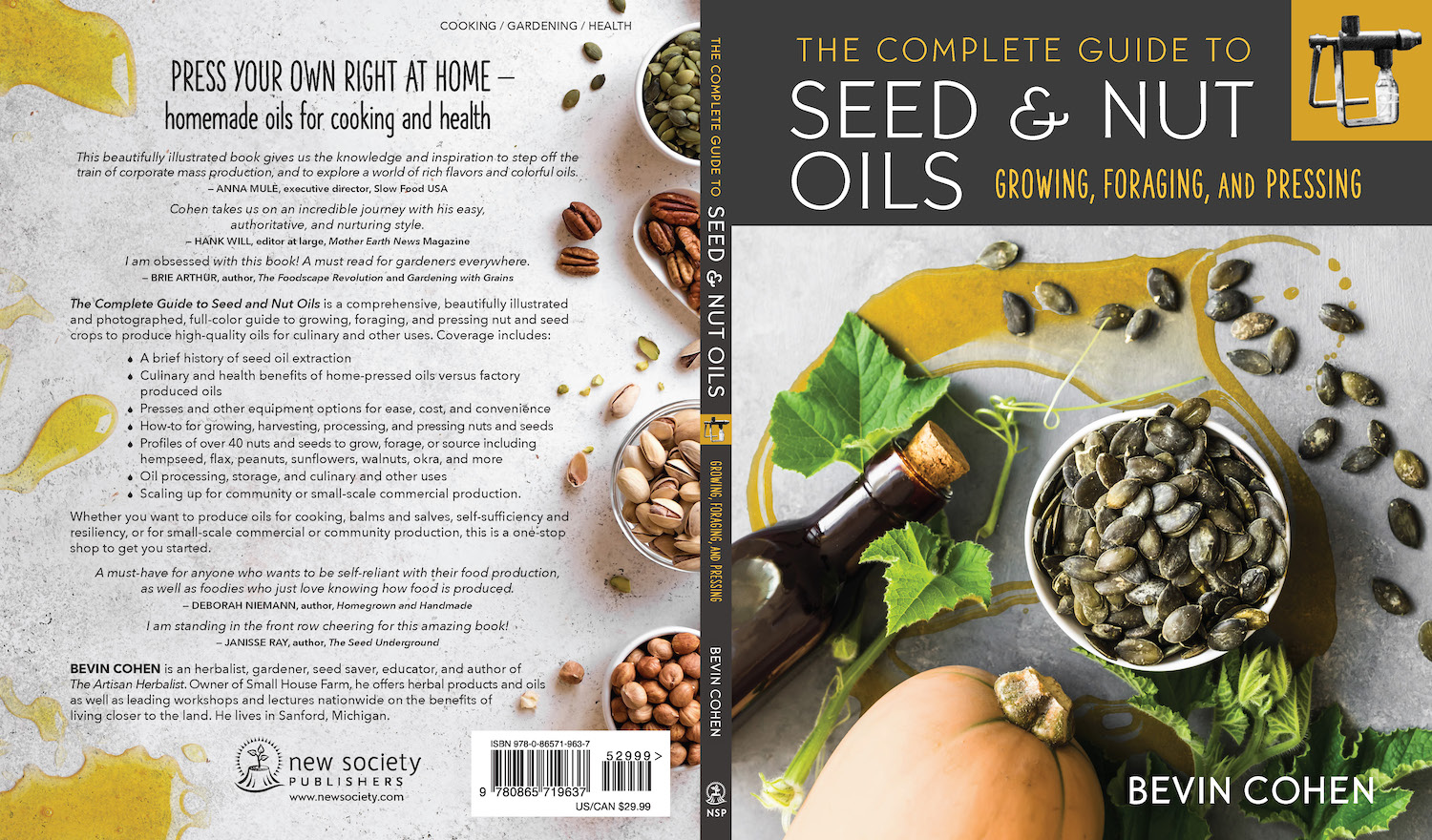The image features the front and back covers of a book displayed against a white background. The book's title, "The Complete Guide to Seed and Nut Oils: Growing, Foraging, and Pressing," is prominently showcased on the right side in alternating gold, white, and yellow lettering against a black backdrop. The front cover includes a detailed, autumnal-themed photograph set on a gray tabletop. This image features a long-necked amber bottle with a natural cork, artfully spilled oil, scattered seeds, green pumpkin leaves, and a white ceramic bowl filled with pumpkin seeds, positioned next to a whole pumpkin. The author's name, Bevan Cohen, is printed in white at the bottom right of the front cover. 

The back cover, shown on the left side, is marked by the phrase "Press Your Own Right at Home" in black lettering, followed by "Homemade Oils for Cooking and Health." A barcode is situated in the bottom right corner. The back features a pattern of spilled yellowish oil and images of several white bowls filled with various nuts, including green nuts, pecans, pistachios, and another type of brown nut. The spine of the book runs down the center of the image, displaying a mix of grays, gold, white, and black colors. New Society is noted as the publisher.